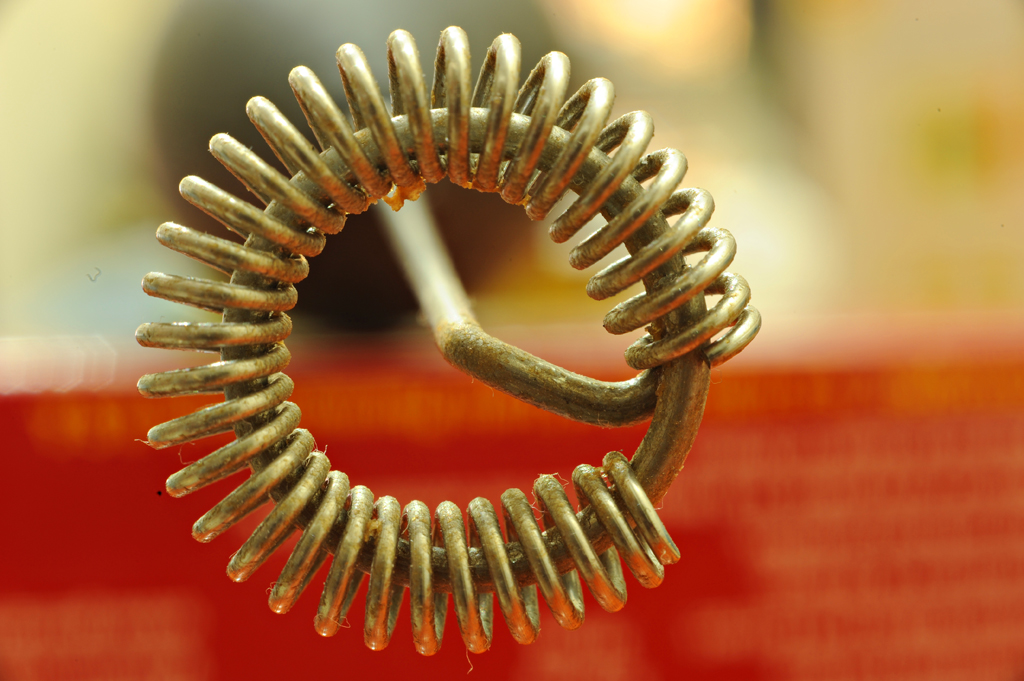The photograph features a detailed close-up of a metallic device, primarily composed of a circular ring with a bronze-colored, tightly wound coil encircling it, giving it the appearance of a spring wrapped around the ring. The coil material appears to be brass, exhibiting a golden hue. Attached to one section of the ring is a curved rod that extends backward and connects to a round black object, possibly a handle or a component meant to rotate the device. The background of the image is distinctly blurred, with the top half displaying yellow with black blobs, reminiscent of a balloon-like shape, and the bottom half presenting as a solid red surface, likely a table. Notable details include signs of dust and grime on the ring, suggesting the device might be an aged or frequently used electrical appliance.